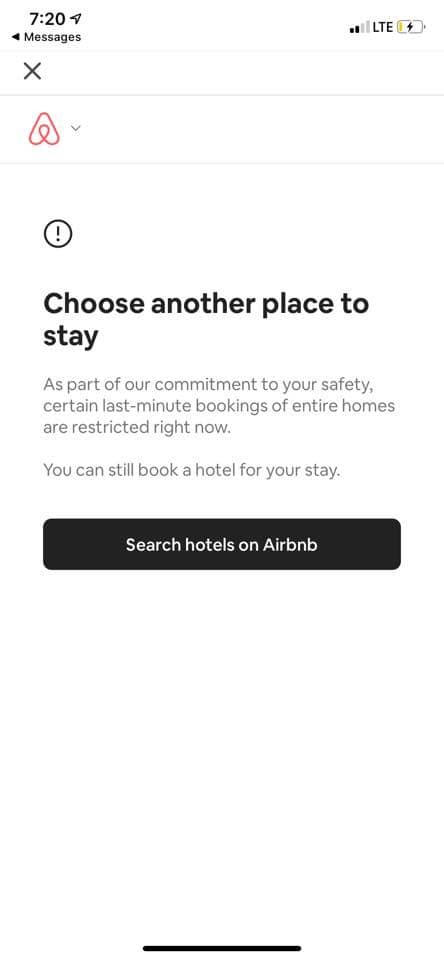**Descriptive Caption:**

"Screenshot captured at 7:20 PM on a smartphone, displaying various phone status indicators. The location-sharing icon is active, showing two out of four cell phone bars. The phone is charging, indicated by a low battery level within battery-saving mode. The data connection is LTE. An unrecognized icon appears at the top left. The topmost left corner features an X button for exiting the page. The main content includes a large exclamation mark inside a circle, accompanied by a message stating, 'Choose another place to stay. As part of our commitment to your safety, certain last-minute bookings of entire homes are restricted right now. You can still book a hotel for your stay. Search hotels on Airbnb.' The text is black, and the message is urging users to find alternative accommodations. The top-left corner showcases the Airbnb logo, which resembles a red triangular shape with a loop. A black button with white text beneath the message reads, 'Search hotels on Airbnb.'"